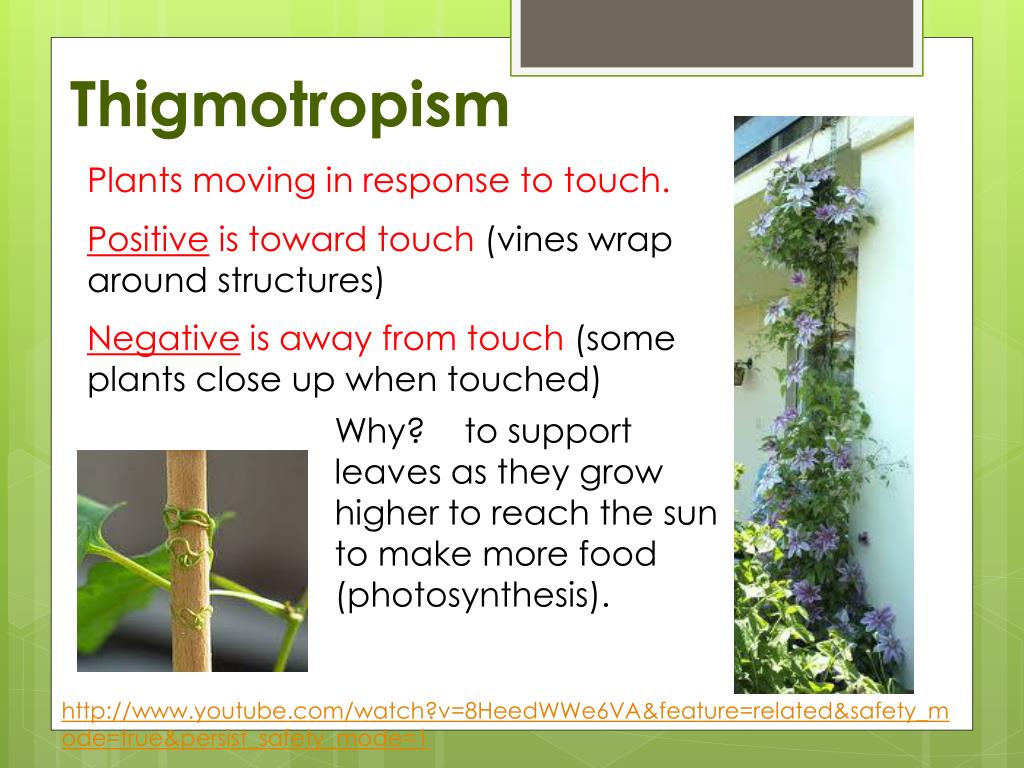The image is a snapshot of a PowerPoint presentation slide with a detailed design and informational content. The outer border transitions from a lighter green in the upper left to a darker green in the lower right. The central area of the slide has a white background, and the title at the top in dark green reads "Thigmotropism." Below the title, in smaller red font, it states, "plants moving in response to touch," with the subsequent description breaking down the concept into finer details. The text explains that a positive thigmotropic response is towards touch, causing vines to wrap around structures, while a negative response is away from touch, noting that some plants close up when touched. It elaborates that this behavior supports leaves as they grow higher to reach sunlight for photosynthesis. Accompanying the text, on the right-hand side, is an image of a vine growing upwards along a balcony, while the lower left corner displays a smaller picture of a vine wrapped around a tree. The slide includes varying colors like green, red, brown, yellow, blue, and purple, and concludes with a link to a YouTube site at the bottom.